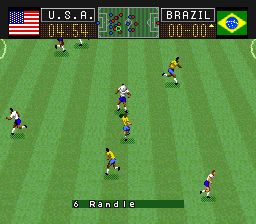The image captures a video game scene of a soccer match on a green field with alternating light and dark green stripes. Players from two different teams are running around: one team wears white shirts and blue shorts, while the other team wears yellow shirts and blue shorts. The player in the center stands out with a helmet, unlike the rest. At the top of the image is a scoreboard with "USA" on the left, showing a score of 4.54 alongside the American flag, which is red, white, and blue with white stars. On the right side of the scoreboard, "Brazil" is noted with a score of 0.00 and accompanied by the Brazilian flag, which features green with a yellow diamond and a blue circle with yellow stars. At the bottom of the image, the text "6 Randall" is displayed in white letters.